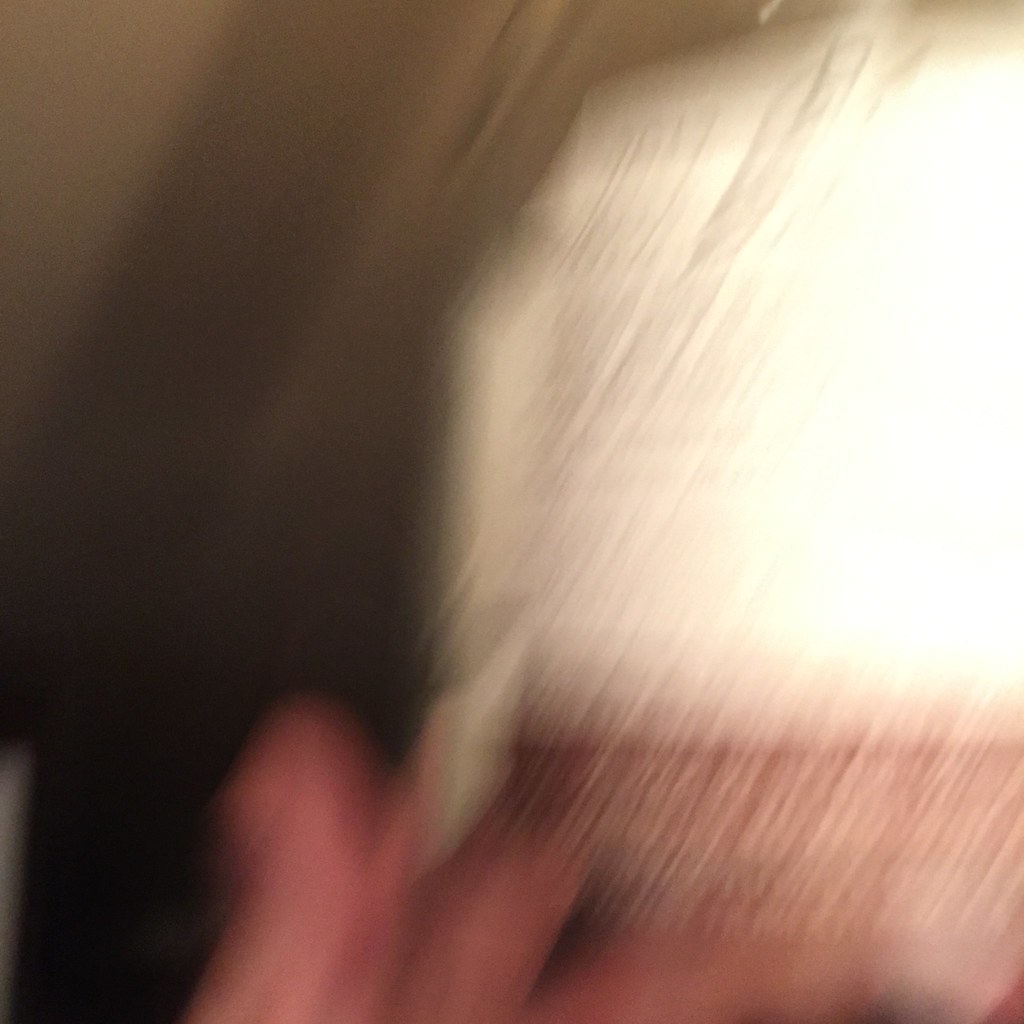This photograph is highly blurred and lacks focus, making it challenging to discern definitive details. It appears to capture the upper portion of a person's face, from just below the eyes to the top of the head. The individual seems to be wearing a white hat or may have gray hair, though this section is significantly obscured by a glaring white flash that suggests overexposure. The person's hand is raised beside their face, though it is also unclear due to the blurriness. The image contains multiple white streaks throughout, contributing to its chaotic appearance. The background on the left side of the photo is a light beige with several dark streaks. The bottom left corner shifts to a considerably darker tone, adding to the overall indistinct and abstract quality of the photo.